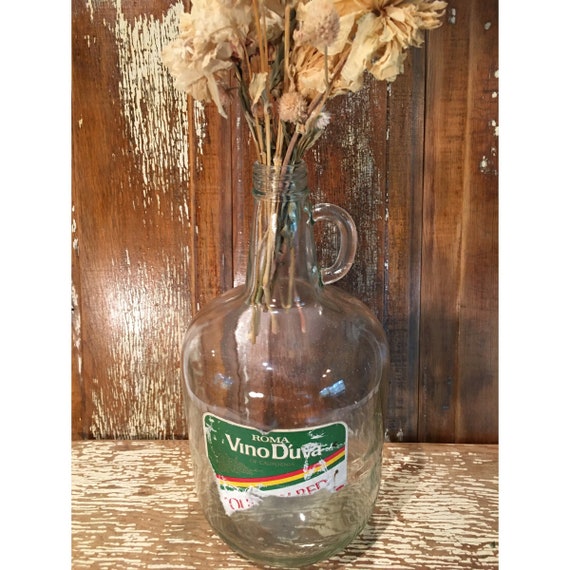The image depicts a large, repurposed glass bottle with a distinctive narrow neck and a semicircle handle on the left side. The body of the bottle transitions from the skinny neck to a wide, bulbous base. A partially torn green and white label on the front reads "Roma Vino," but the bottom of the label is missing, obscuring some text. Inside the bottle, a collection of beige, fluffy plants and brown sticks, resembling dried flowers or wheat, emerges from the top. The background consists of a wooden surface and a wooden wall, both showing scratch marks. The setting is bright and well-lit, with a clear and detailed view of the objects.